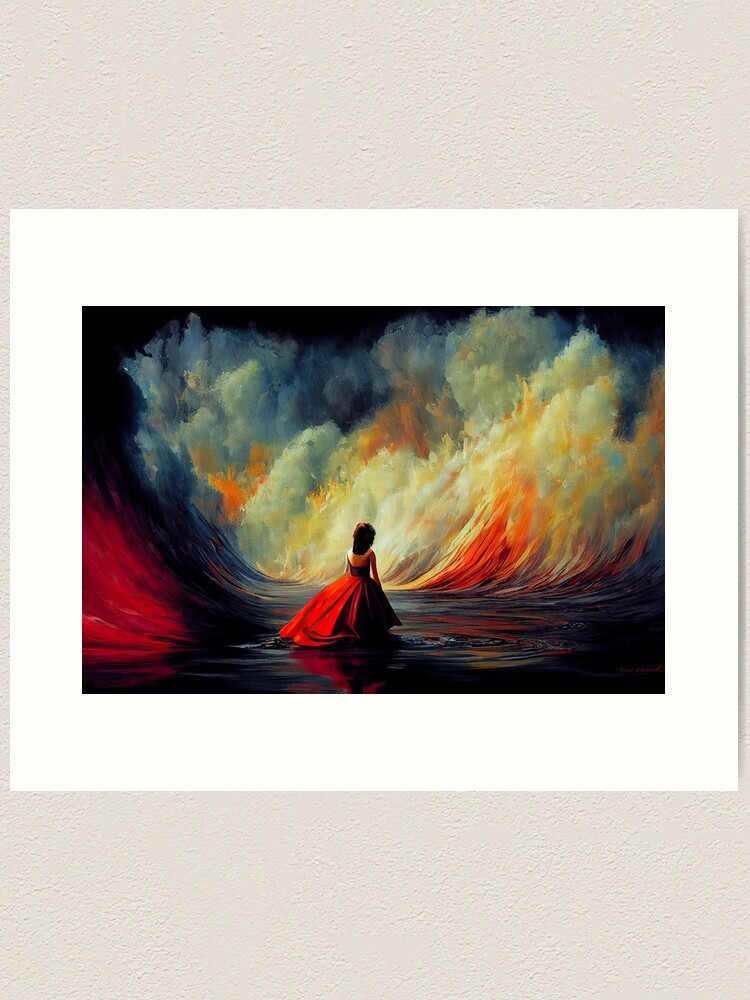This is a detailed image described through different perspectives. The photograph or painting, rendered in watercolor, features a vertical rectangular format. At its center is a smaller, white horizontal rectangle that serves as matting for the artwork inside. The subject of the painting is a woman in a striking red ball gown with a voluminous skirt and what appears to be either shoulder straps or a strapless design. Her long dark hair cascades down, and she is positioned looking away, drawing the viewer's gaze towards the back of the scene.

The setting around her is somewhat ambiguous and abstract. The ground she stands on is dark and curls upward at the sides, transitioning into a vibrant palette of reds and oranges. In front of her, there's an interplay of white and colored elements that resemble smoke, clouds, or perhaps the crests of waves. These elements exhibit a mix of orange and blue hues, creating a surreal, ethereal landscape. Behind her, more red, like reflected light, appears on what could be a cliff, adding to the dynamic and somewhat dream-like quality of the scene. The overall impression is one of vivid color contrasts and an almost mystical atmosphere.